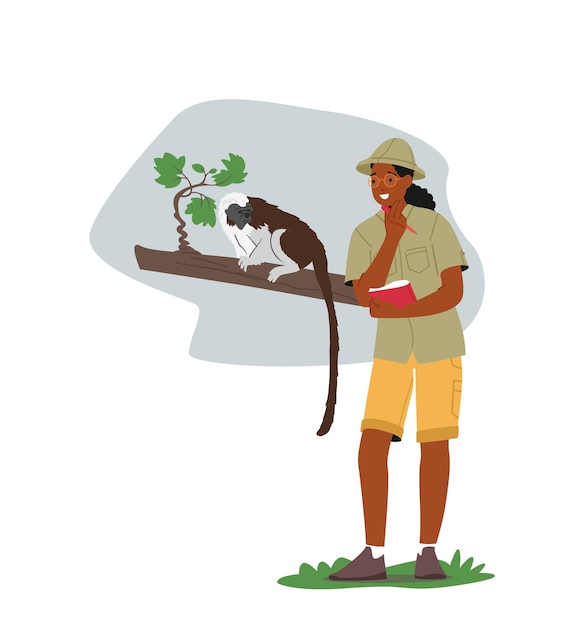This digital clipart image features a simplified, color drawing of a stereotypical female scientist or zookeeper observing an animal in the wild. The scientist has dark skin and black hair styled in a ponytail, and she wears a tan safari hat and red glasses. Her attire includes a tan button-up shirt with chest pockets, yellow cargo shorts, white ankle socks, and black shoes. Standing on a small tuft of grass with three blades on either side of her, she holds a pink notebook with a pen against her middle using her left arm while her right hand is positioned under her chin in a quizzical pose, suggesting deep thought.

In the background, a blue-shaded area from her waist up highlights a log extending from behind her to the left. The log, missing its tree, appears almost as if it is protruding from her back. A large branch on this log features three prominent leaves and a smaller sprout of leaves. Positioned on the branch close to the scientist is a lemur-like creature with white fur on its head and chest, black fur on its back, and gray limbs. Its exceptionally long black tail dangles off the branch. The lemur's head is tilted towards the right, appearing as if it is looking backward over its shoulder at the scientist. The overall drawing is simplistic, focusing more on conveying a scene of observation and study, despite leaving some elements abstract and open to interpretation.